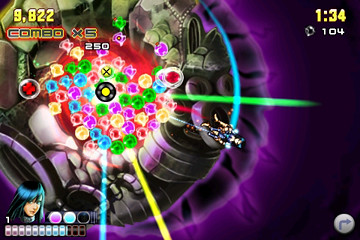The image depicts a 2D video game scene featuring a small ship positioned centrally, engaged in combat. The player appears to be firing towards a central area populated with various colorful icons, including hues of purple, blue, red, and yellow. At the core of this cluster is a black circle with a yellow center, situated within what seems like a pit. Above this central cluster, a yellow icon with a cross or an "X" shape is visible. 

The game's environment has a robotic or mechanical aesthetic, characterized by a grayish area surrounding the main elements. To the top left of the screen, the user interface (UI) displays a score of 9822, a combo multiplier of 5, and an additional score of 250. The bottom left corner features an image reminiscent of an anime character, adorned with various small markers and colors. The top right corner shows a timer reading 134 seconds, followed by another value of 104. Finally, the bottom right corner contains an arrow icon, likely indicating an action or direction for the player.